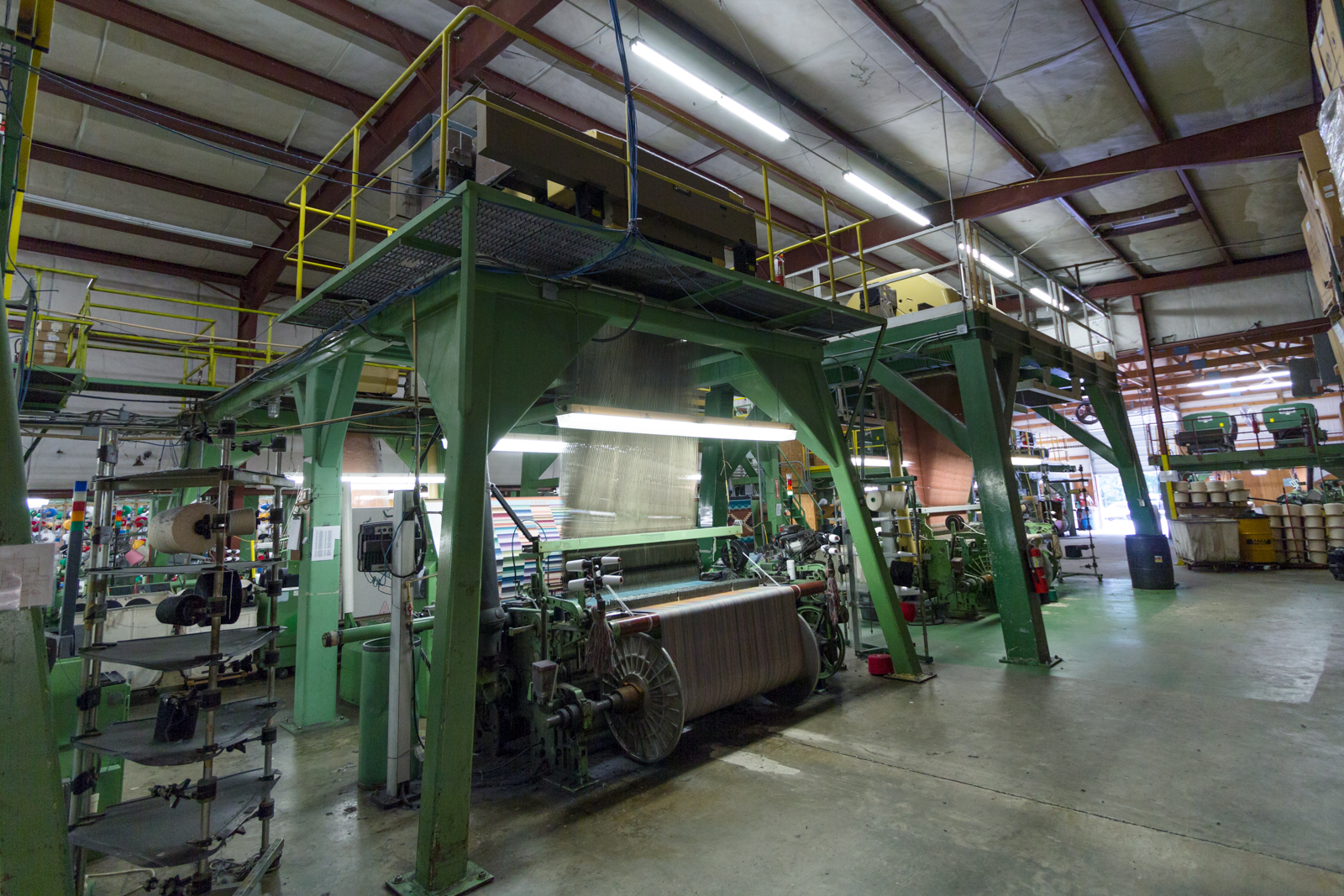In this detailed image of an industrial manufacturing plant, we observe a spacious area characterized by burgundy-framed metal structures supporting a white ceiling, complemented by white walls and a gray cement floor. Dominating the scene are two large green platforms with sturdy metal legs. Atop these platforms are intricate bases equipped with yellow and silver railings, designed for personnel access. Below, a complex machine that resembles a loom or feeder mechanism processes material. This machine features a prominent spindle on the ground, guiding a large, flat sheet of material upward through various rollers, suggesting it's feeding or weaving fabric. Behind this setup, there is an array of colored fabrics and various materials stored on metal shelving, hinting at the diverse manufacturing activities conducted in this well-equipped facility. The open ceiling with visible beams and insulation adds to the industrial ambiance of the scene.